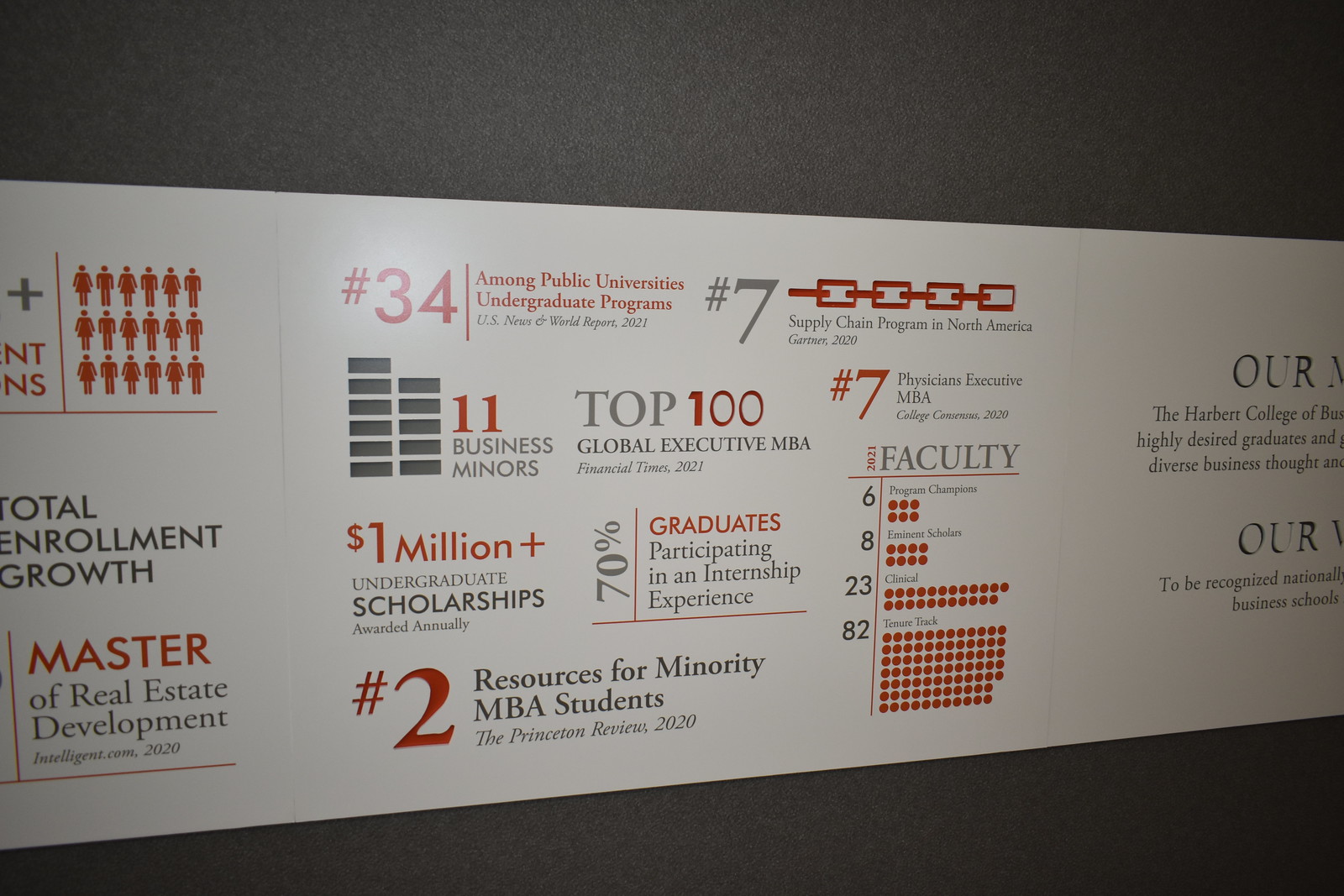This image features a color photograph of a white poster banner mounted against a grayish-black background, creating a stark contrast. The banner, designed in landscape orientation, spans horizontally from the left to the right side of the image. It presents several highlighted achievements and statistics of an unspecified MBA program, particularly focusing on its supply chain and executive MBA offerings. Key details include the program's ranking as the number seven supply chain program in North America and its distinction as the number seven physician executive MBA. Additionally, the program is recognized as the number two resource for minority MBA students by the Princeton Review and is ranked number 34 among public universities' undergraduate programs.

The banner also features notable accomplishments like awarding one million dollars in undergraduate scholarships annually and having 70% of graduates participate in internship experiences. The design includes color writing primarily in red and gray, with bold red numbers highlighting various ranks and metrics. On the left side of the banner, images of men and women are visible, along with a bar graph detailing the faculty distribution across different subjects. Other notable terms include "total enrollment growth" and "11 business minors." Although the specific college name is not mentioned, the banner conveys the program's prestige and commitment to academic excellence.